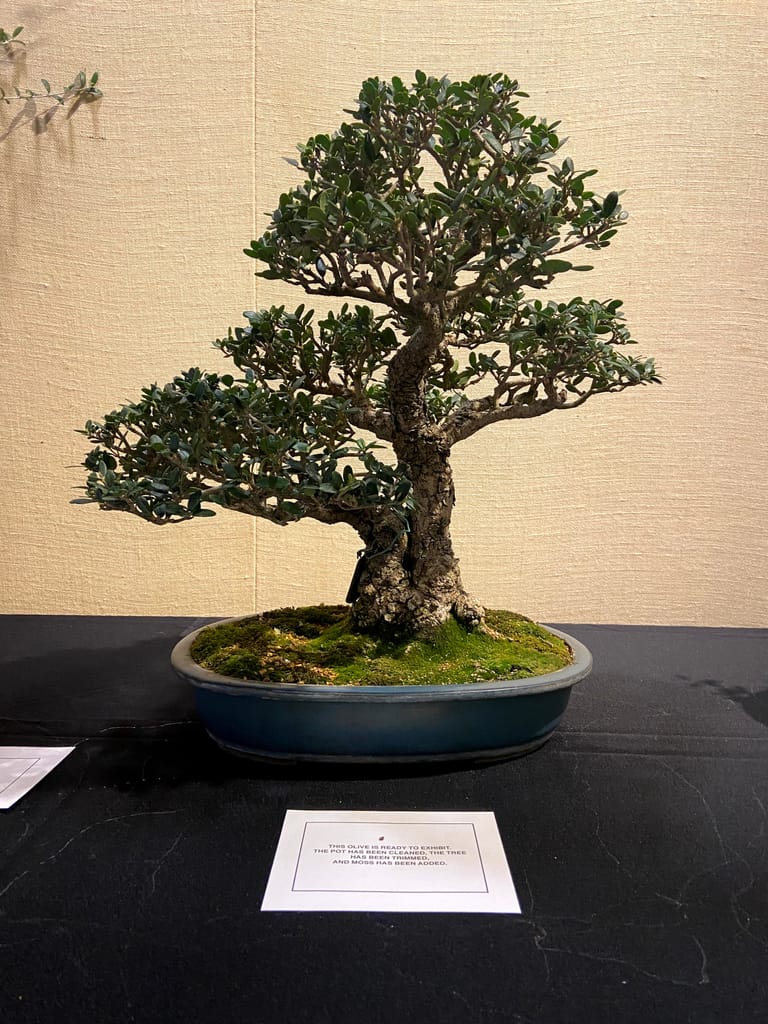The image features an elegant bonsai tree displayed centrally on a black tabletop, which occupies the bottom third of the picture. The table holds a white placard with unreadable text. The bonsai tree is planted in an oval-shaped, shallow blue bowl filled with lush green moss that resembles grass. The tree itself is notable for its double trunk: the right trunk grows straight up, extending vertically with smaller branches, while the left trunk bends sharply at a 90-degree angle, reaching out horizontally before ascending slightly. The sturdy trunks, characterized by shades of dark and light brown, support a canopy of small, dark green leaves lightly tinged with white. The upper two-thirds of the image reveal a pinkish-beige, textured wall, which could indicate a museum or garden setting. A branch from another tree intrudes from the top right corner, adding to the natural feel of the scene.